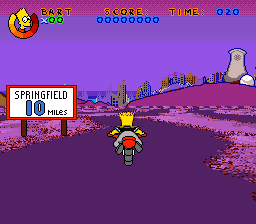A vivid screen capture from a Simpsons video game showcases Bart Simpson prominently in the upper left corner, beside a fully colored health meter indicating optimal health. The meter transitions from yellow to dark red, demonstrating Bart's unscathed condition. The overlay shows "Bart x 000" in green and "4000" in blue, alongside a timer counting down from 20 seconds. Bart is depicted riding a motorcycle along a whimsical purple path. A road sign on the left reads "Springfield 10 miles" with the '10' in blue and the rest in black. The iconic Springfield Nuclear Power Plant is visible on the right, with the cityscape of Springfield stretching out in the background, setting a familiar and immersive scene.